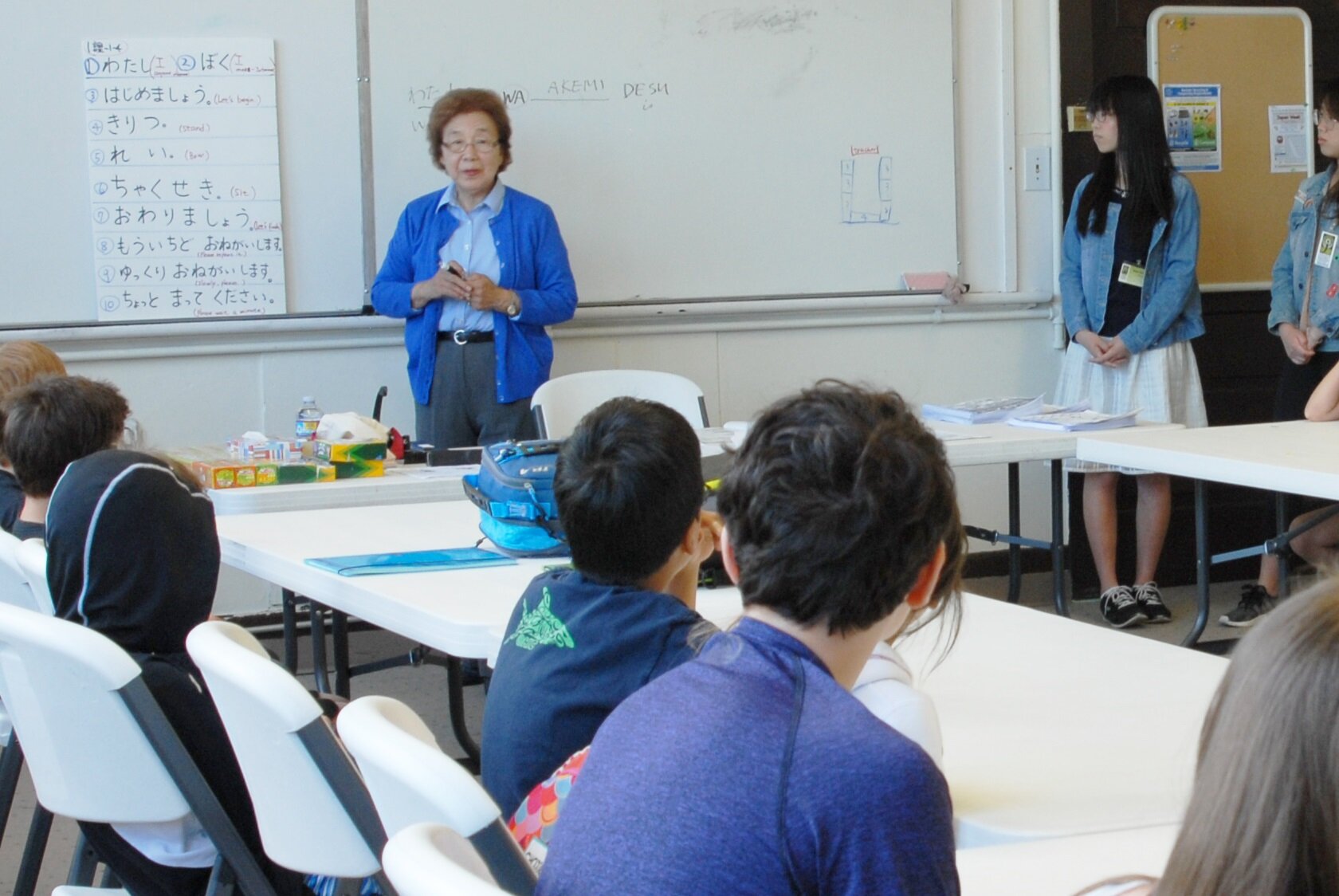In this detailed photograph of a classroom, an Asian woman—likely the teacher—is seen standing in front of a whiteboard adorned with Asian characters, possibly suggesting the setting is a Japanese or Chinese class. She is wearing a blue cardigan over a blue collared shirt, accessorized with a black belt and grey pants. Her hands are outstretched as she engages with the students, and she is wearing glasses. 

The classroom features white walls, a whiteboard, and white tables where multiple students are seated. These students, mostly with black hair and appearing to be of Asian descent, are attentively watching the teacher. One student in a black jacket has their hood up, while another in the corner has long, light brown hair. On the far right, there are two girls standing near the teacher. One girl is in a blue long-sleeved shirt with a black shirt underneath and a white skirt paired with black tennis shoes. The second girl has long black hair and is dressed in a blue jean jacket.

Crayon boxes and markers are scattered across the table in front of the teacher, suggesting a creative activity. The overall scene reveals a lively and engaged classroom with clean, organized tables and a door visible to the far right.